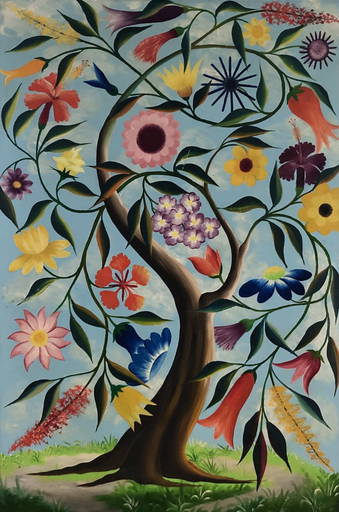This painting, titled "Orbre au Papillon" by Haitian artist André Pierre, features a vividly abstract depiction of a towering tree rooted in lush, green grass. The tree, with its twisting and swirling main branches, commands the center of the composition. The primary branch arcs to the right before looping back to the left, while a secondary branch splits off and swirls to the right, each adorned with vibrant foliage. The focal point of the painting is the explosion of diverse and colorful flowers that bloom from these branches. These flowers, resembling sunflowers, irises, hyacinths, and lilies among others, showcase a spectrum of colors including pink, yellow, orange, blue, purple, red, and black. The tree's bark is textured with various shadows, enhancing its dimensionality against a backdrop of a clear blue sky dotted with light clouds. The scene conveys a sense of abundant life and natural beauty through its dynamic composition and rich use of color.